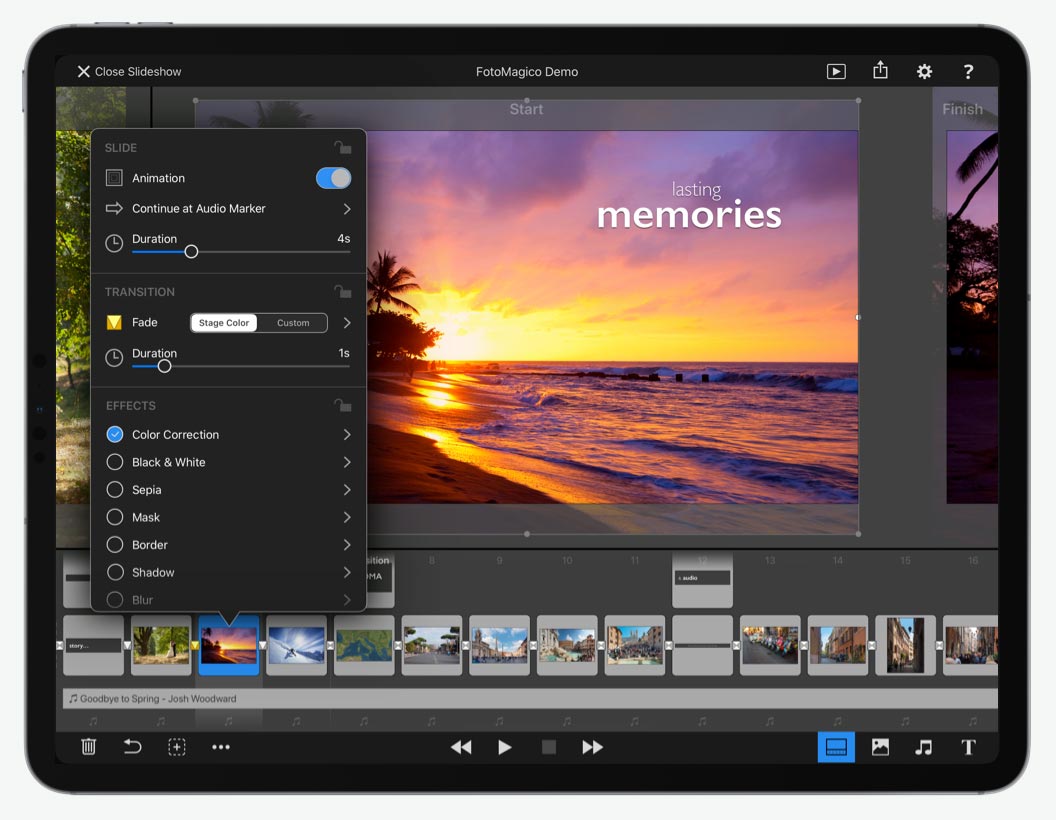The image features a tablet displaying an application interface, framed by the device's black border and visible hardware buttons. On the screen, a detailed menu of the app's settings is open, presenting options in a sleek black background with white text. The settings list begins with "Animation" and includes options such as "Continue at audio marker" and "Duration." Further down, under the "Transition" category, "Fade" and "Duration" are listed. The "Effects" section includes choices like "Color Correction," "Black and White," "Sepia," "Mask," "Border," "Shadow," and "Blur," indicating comprehensive photo or video editing capabilities.

At the top of the interface, the application is identified as "Photo Magico Demo," suggesting it is a trial version of a photo editing or presentation software. Example images are also prominent on the screen, including a tranquil beach scene with the water reflecting a picturesque sunset. Superimposed on this image, the text "Lasting Memories" is elegantly written in white. The combination of the interface details and sample images provides a clear indication of the app's functionalities and user interface.